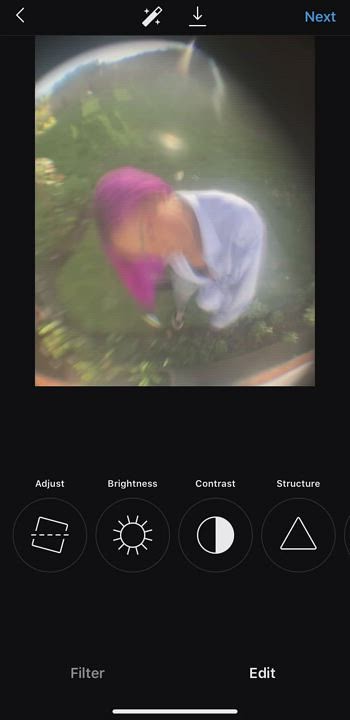The image depicts a smartphone screen displaying a photo editing interface. Dominating the screen is a blurry, overhead shot of a girl with purple or pink hair, wearing a white shirt or jacket, seemingly in a garden surrounded by foliage. Key interface elements are visible: at the top left, a white arrow points to the left alongside a stick icon with stars and a downward arrow, while the top right features the word "Next" in blue. Below the photo, there are four grey circles, each containing white icons representing different editing options labeled "Adjust," "Brightness," "Contrast," and "Structure." At the bottom left of the screen is the word "Filter" in white, and on the bottom right, a bolder white "Edit."